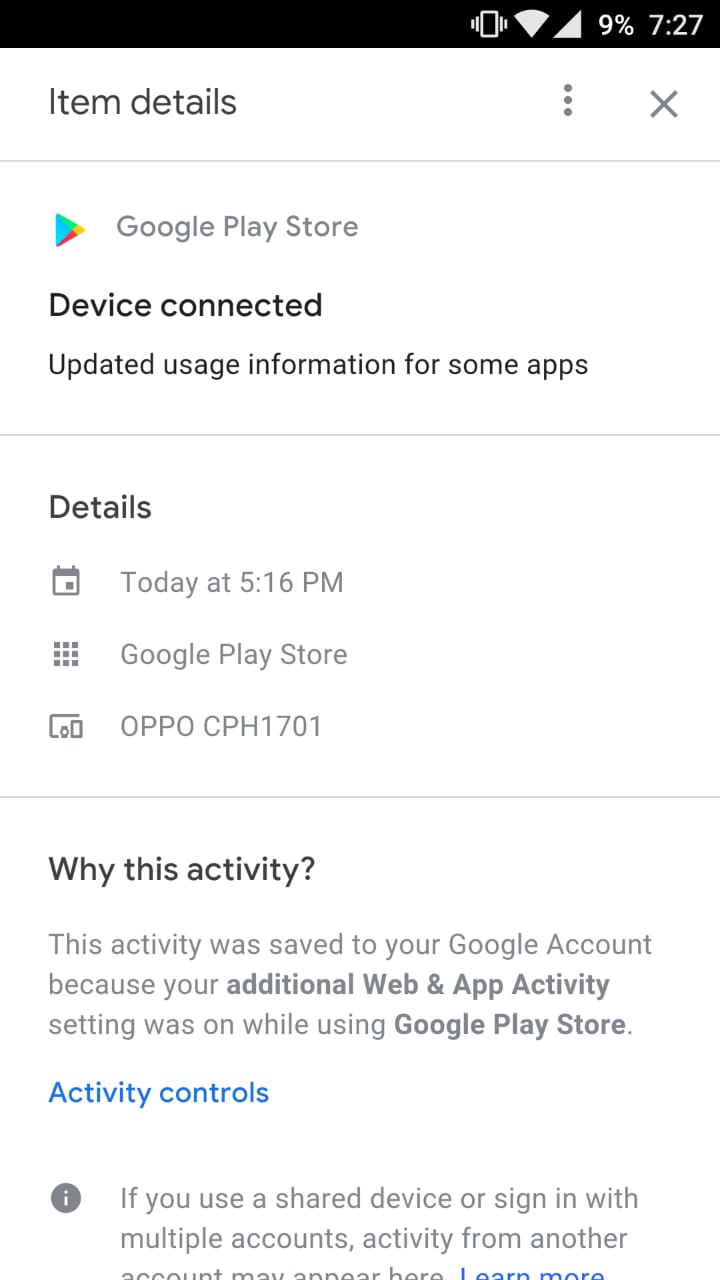This is a detailed screenshot from the Google Play Store. At the top, a black bar displays various status icons: vibration mode is on, Wi-Fi is at full strength, full signal bars, only 9% battery remaining, and the time is 7:27. Below the black bar, the interface shows a white section with "Item details" on the left, a vertical three-dot menu in the center, and an 'X' close button on the far right. A thin gray line separates this from the content below.

The next section features the Google Play Store icon—a right-facing triangle composed of overlapping blue, green, yellow, and red shapes—next to the text "Google Play Store" in light green. Beneath that, in black text, it says "Device connected". Below this, the message "Updated usage information for some apps" appears, followed by another thin gray line.

The section labeled "Details" is presented in black text. It includes icons: a calendar, a nine-square grid, and a multi-screen format for devices like screens, tablets, and phones. Next to these icons, it states:
- "Today at 5:16 p.m." for the calendar,
- "Google Play Store" for the grid icon,
- "OPPO CPH 1701" for the multi-screen icon, all in light gray.

Another gray bar separates the next part, where "Why this activity" is shown in black text. Below it, in gray text, it reads: "This activity was saved to your Google account because your additional web and app activity setting was on while using" with "Google Play Store" repeated in darker gray. At the bottom, in blue text, the link "Activity controls" is displayed next to an information icon. This section notes: "If you use a shared device or sign in with multiple accounts, activity from another", but the third line is cut off, indicating it likely says, "account may appear here". The phrase "Learn more" is also in blue.

This screenshot captures various elements and information regarding activity tracking linked to the Google Play Store on a device.